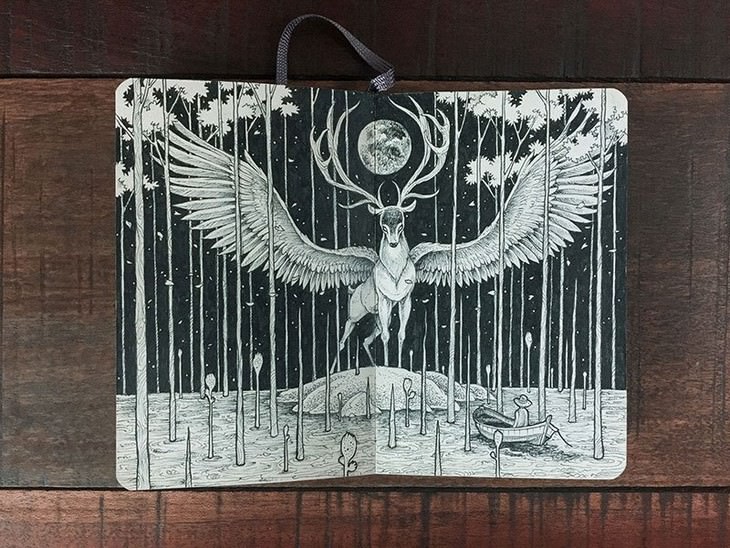The image is a highly detailed, artistic black-and-white drawing that resembles a charcoal sketch. It portrays a mystical scene centered around a gigantic, 30-foot tall deer with expansive angel wings, standing majestically on a small island in the middle of a tranquil pool of water. This fantastical deer has enormous antlers, which encircle the moon and dominate the night sky filled with starry white blotches. The stag’s eyes are eerily whited out, and its antlers are adorned with numerous points.

Surrounding the water are shoots of plants, some taller than the deer, as well as slender trees with pencil-thin trunks and foliage perched at their tops. A small rowboat, carrying a lone person wearing a straw hat, sits in the bottom right corner of the scene, the individual gazing up at the imposing deer.

The drawing rests on a dark, polished wooden surface, either a table or floor, characterized by stained panels with visible joints. The artwork itself appears to be on foldable cardboard with a carrying strap, some dots scattered across it, hinting at texture and dimension, and it conveys an otherworldly atmosphere with both natural and surreal elements intertwined.